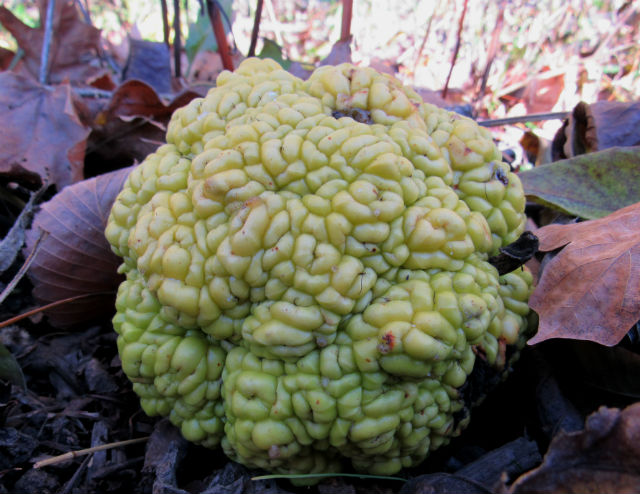The image is a detailed, close-up color photograph taken in a forested area. It captures various forms of ground debris such as dried fallen leaves, sticks, and plant stems. Dominating the center of the composition is a mysterious round cluster, possibly biological in nature, with light yellow, kidney-shaped nodules that form a complex, curvy structure resembling a cauliflower head. The surrounding leaves display a spectrum of colors, including reddish-orange and dark green, creating a vivid contrast with the cluster. The scene is sunlit, suggesting a clear day, with dappled light enhancing the realism of the organic surroundings. The photo is free from any text or people, focusing purely on this intriguing natural formation amidst the forest floor.